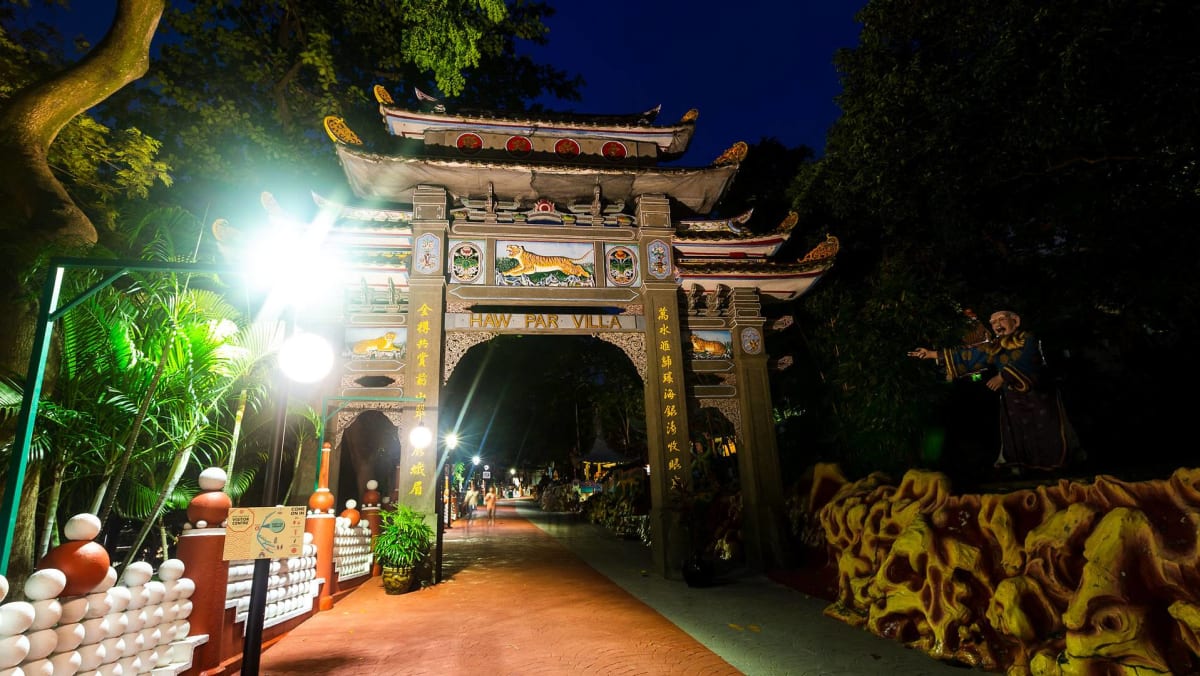The image captures the nighttime entrance of Haw Par Villa, a thematic park displaying Chinese architecture. Dominating the center is a grand, multi-tiered archway with a pagoda-style roof, accentuated by brown arches with cyan details. This arch features intricate design elements, including two tigers flanking a central emblem. Written in orange text, "Haw Par Villa" is prominently displayed at the top of the arch. In the foreground, an orange path leads under the arch toward distant figures and small buildings, punctuated by a small potted plant and a map stand.

To the left of the archway is a traditional Chinese fence composed of alternating white balls and red posts, illuminated by bright street lamps. The right side of the arch is marked by a lifelike statue of a man in a blue and beige robe, seemingly gesturing to welcome visitors. This figure stands against a complex, wavy stone wall in shades of beige and brown.

Surrounding the entrance, verdant trees and various greenery add a natural frame to the scene, while the night sky in dark blue provides a dramatic backdrop. The overall blend of lighting and architectural elements exudes a welcoming yet mysterious ambiance, inviting visitors to explore further.